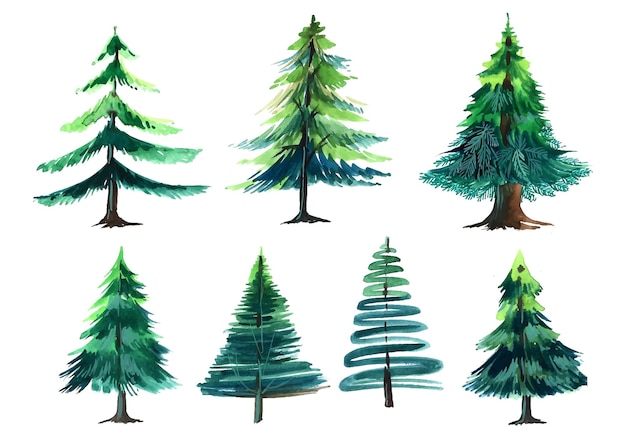The image showcases seven detailed digital drawings of evergreen and pine trees, organized in two rows, with the top row comprising three trees and the bottom row four. This practice exercise highlights different artistic styles and techniques used to depict these familiar trees.

- **Top Row:**
  1. The **leftmost tree** features downward and outward sloping leaves with varying shades of green, possibly watercolor with hints of mixed media, painted on a thick, brown trunk.
  2. The **middle tree** is fuller, resembling a classic Christmas tree, with a symmetrical triangular shape and multi-tonal green leaves that lighten towards the top, indicating the effect of sunlight.
  3. The **rightmost tree** boasts a notably thick, dark brown trunk and cascading dark and light green leaves, creating a dense, heavy appearance.

- **Bottom Row:**
  1. The **leftmost tree** mirrors the Christmas tree style from the top row, with its pointed triangular shape and consistent green foliage.
  2. The **second tree** has visible branches interspersed within swirled leaves, showcasing a mix of green hues through a brush-stroke technique.
  3. The **third tree** displays a straightforward, rough representation using brown branches and simple green squiggles to form the tree shape.
  4. The **rightmost tree** features leaves that slope downwards, similar in style to the top left tree, continuing the thematic green and brown palette.

Overall, these detailed digital drawings of evergreen and pine trees exhibit a variety of artistic interpretations, primarily using shades of green and brown against a clean, white background. Each tree offers a unique take on this iconic natural form.